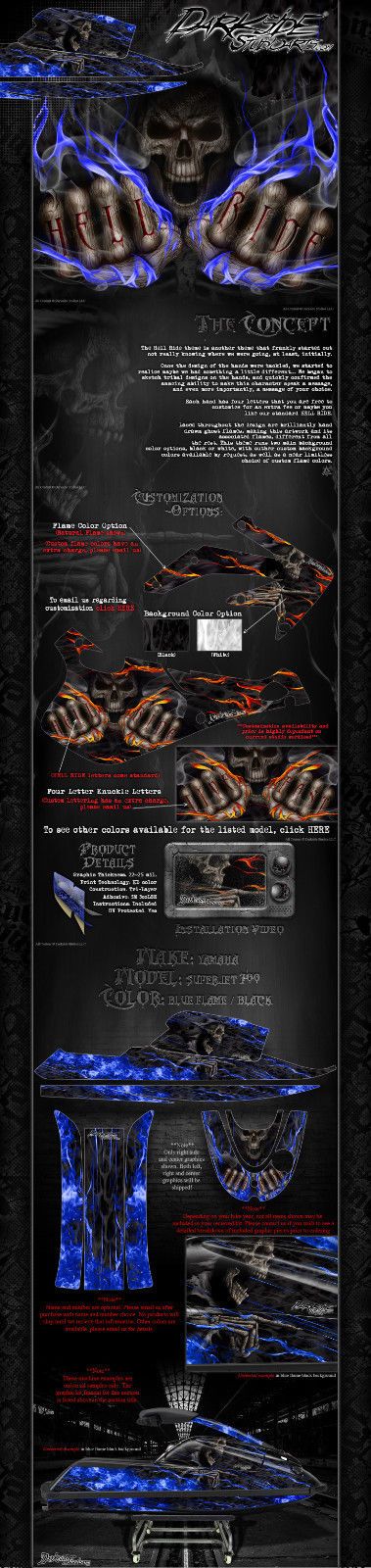The image appears to be a long rectangular concept art for a horror-themed character or advertisement, primarily utilizing a dark black and gray background with vivid accents of blue, red, orange, and white. At the very top, there is a menacing, cartoonish skull character reminiscent of the Grim Reaper, with a hood over its head, holding up its fists enveloped in blue fire. The knuckles display the phrase "Hell Ride" in red text. Just below this, the same skeleton figure is depicted, but now the fire surrounding its hands is red and orange. Further down, the same color scheme of blue reappears, and it looks like the figure might be sitting down or in a car, though it's ambiguous. The entire strip includes numerous smaller white and red text segments, mostly too small to discern. Flanking the skulls and hands are effects of electrified purple lighting accentuating their positions. The design encapsulates a dark, edgy, and supernatural atmosphere, reinforced by the repeated motifs of flaming skeletal hands and skulls, underscored by an unsettling use of vibrant colors against the somber backdrop.